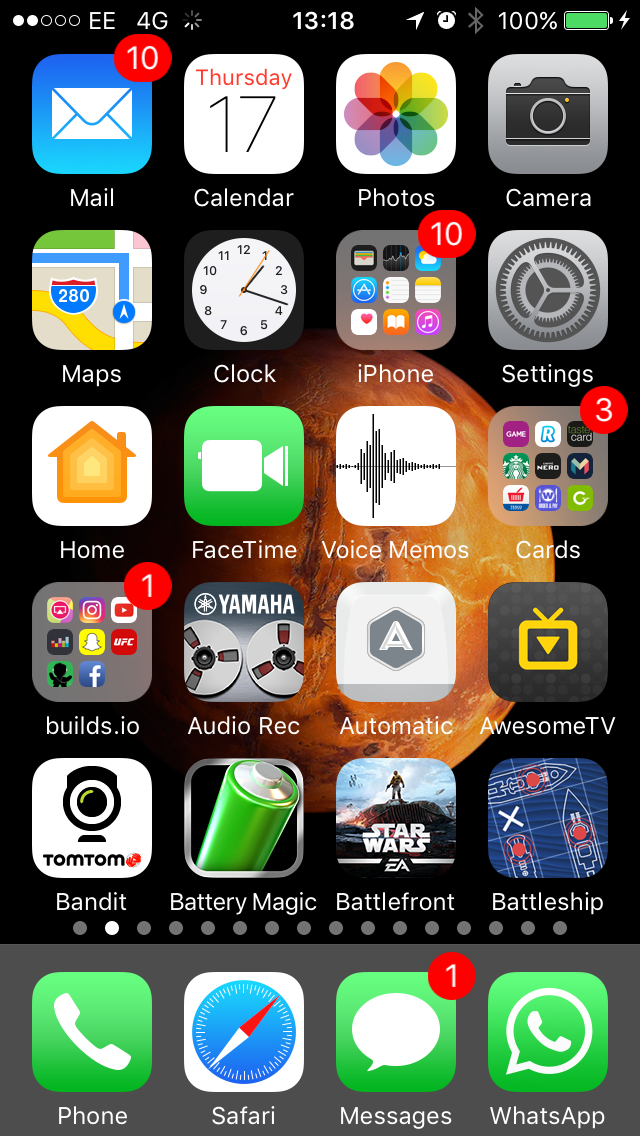The image showcases the home screen of an iPhone, displaying a variety of apps organized in a grid format. 

- **Top Row:**
  - **Mail App:** Icon with a blue background featuring a white envelope, accompanied by a red notification badge displaying the number '10'.
  - **Calendar App:** A white square icon displaying "Thursday" in red text and "17" in black.
  - **Photos App:** Icon featuring a multicolored flower against a white background, representing the colors of the rainbow.
  - **Camera App:** A simplistic black icon of a camera on a gray background.

- **Second Row:**
  - **Maps App:** A stylized map icon with blue, red, tan, and yellow elements.
  - **Clock App:** Icon showing a white clock face with the hands pointing to approximately 1:15.
  - **Folder:** A collection of nine mini-icons representing apps including Wallet, Stocks, Weather, Apple, Notes, Reminders, Health, Books, and Music.
  - **Settings App:** Icon depicted with a gear in gray and black tones.

- **Third Row:**
  - **Home App:** Icon with an orange house on a white background.
  - **FaceTime App:** Green square icon featuring a white camera.
  - **Voice Memos App:** White icon with a black waveform, depicting recorded audio.
  - **Folder:** Another mini-folder with various app icons.

- **Fourth Row:**
  - **Folder:** Contains six smaller app icons and displays a notification badge with the number '1'.
  - **Yamaha Recording App:** A specific app related to Yamaha recording equipment.
  - **A Automatic App:** Likely an app related to automotive or driving assistance.
  - **Awesome TV App:** An app likely related to television streaming or remote control features.

- **Fifth Row:**
  - **TomTom Bandit App:** An app related to TomTom’s Bandit action camera.
  - **Battery Magic App:** An app likely for battery management.
  - **Star Wars Battlefront App:** An app related to the Star Wars Battlefront game.
  - **Battleship App:** An app version of the classic Battleship game.

- **Dock (Bottom Row):**
  - **Phone App:** A green icon with a white telephone receiver.
  - **Safari App:** An icon depicting a compass on a blue background.
  - **Messages App:** A green icon with a white speech bubble.
  - **WhatsApp:** A green icon featuring a white speech bubble and telephone receiver.

Each row carefully arranges apps for convenient access, blending productivity tools, entertainment, and utilities.